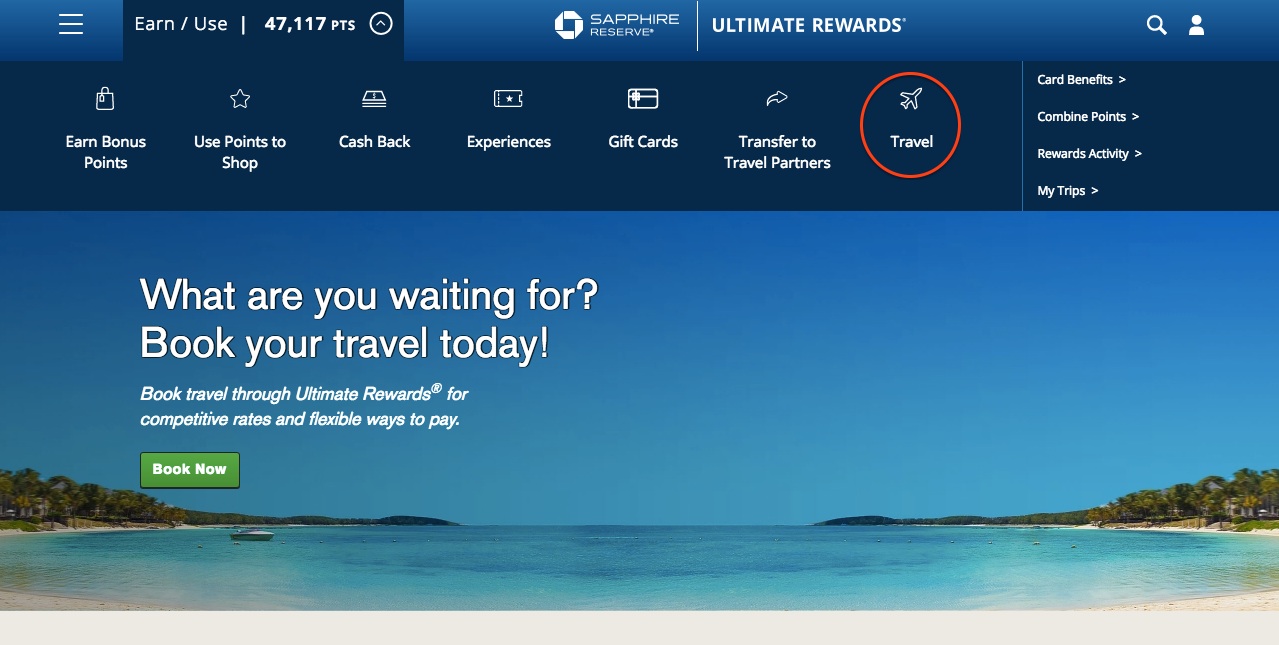The screenshot of a travel website is horizontally rectangular in shape, capturing a scenic background image of a vast body of water flanked by gentle hill-like formations on both the right and left sides. The sky above is a deep, clear blue, adding to the tranquil setting. At the top of the website, a banner displays various elements including the text "Earn Use," a points balance of "47,117 points," the "Sapphire Reserve" logo, "Ultimate Rewards," a search button, and profile icons. 

Beneath this top section, there is a dark blue horizontal banner featuring navigation options such as "Earn Bonus Points," "Use Points to Shop," "Cash Back," "Experiences," "Gift Cards," "Transfer to Travel Partners," and "Travel," with the "Travel" option highlighted by a red circle. 

To the right of this banner, a short vertical list includes links labeled "Card Benefits," "Combined Points," "Rewards Activities," and "My Trips." Dominating the center-left of the image overlaying the scenic background, bold large print reads, "What are you waiting for? Book your travel today. Book travel through Ultimate Rewards for competitive rates and flexible ways to pay," accompanied by a prominent green "Book Now" button. This setup encourages users to utilize their reward points for travel purposes, blending both inspiring visuals and actionable information seamlessly.